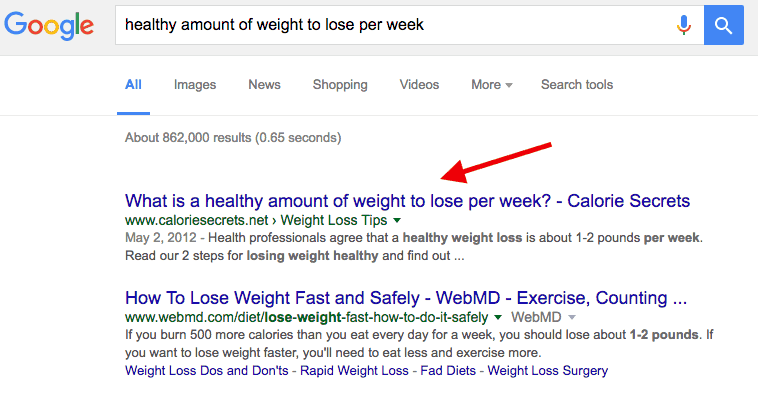The image depicts a web search results page with typical elements found in a modern web browser screen. In the upper right-hand corner, familiar icons in blue, red, yellow, and green are visible, likely representing a well-known search engine. The search query entered is "healthy amount of weight to lose per week."

To the right of the search bar, there are icons for a microphone and a search button. The top navigation bar offers options like "All," "Images," "News," "Shopping," "Videos," and "More," with a pull-down menu and search tools available. The search has returned about 862,000 results in approximately 0.5 seconds.

At the very top of the search results, a red arrow highlights the first entry titled "What is a healthy amount of weight to lose per week?" from caloriesecrets.net. This site is listed under the categories "weight-loss tips" with a dropdown menu for further options. The second result is from WebMD, titled "How to lose weight fast and safely," categorized under "exercise," "counting," and accessible through webmd.com/diet/lose-weight, focusing on safe weight loss practices.

Each search result includes black-text descriptions detailing content from the respective websites. Both highlighted results recommend a weight loss of one to two pounds per week. Links to the websites are displayed in blue text, while the URLs are in green text, consistent with standard search result formatting.